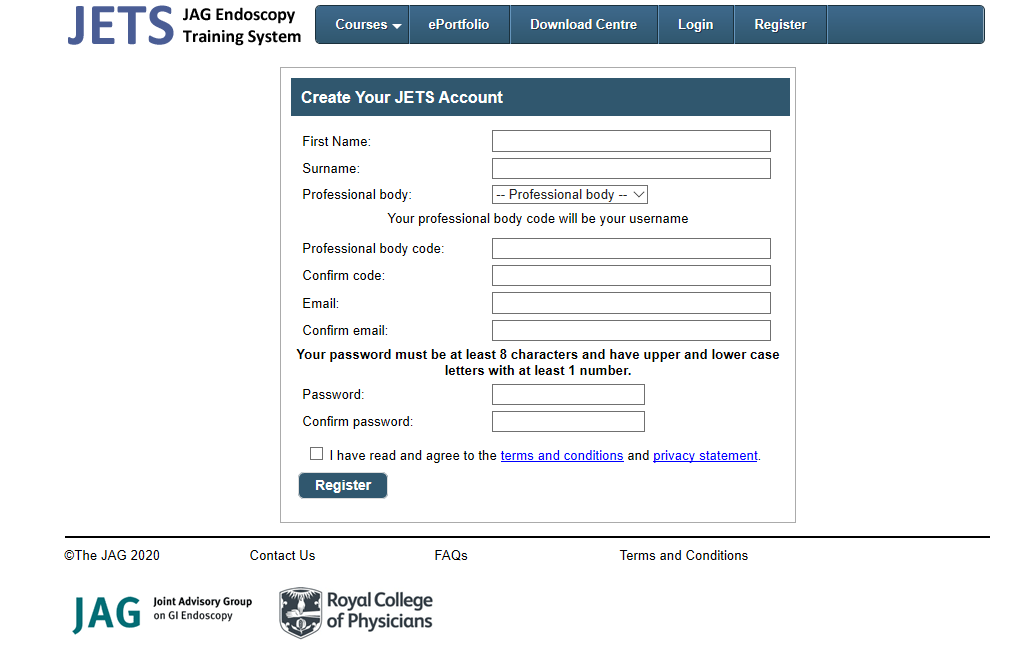The image depicts a webpage from the JETS JAG Endoscopy Training System. 

At the top of the page, there is a bluish rectangular header featuring several navigation tabs. These tabs include "Courses" (with a drop-down arrow), "ePortfolio," "Download Center," "Login," and "Register." 

Dominating the center of the page is a large square section titled "Create Your JETS Account." This area contains several labeled text boxes for users to enter their details: First Name, Surname, Professional Body (with a drop-down menu), Professional Body Code (noting this will be the username), Confirm Code, Email, Confirm Email, Password, and Confirm Password. There is a note specifying that passwords must be at least eight characters long and include both uppercase and lowercase letters, as well as at least one number.

Below the text boxes, there is a checkbox accompanied by the statement "I have read and agreed to the terms and conditions and privacy statement," with the terms and conditions and privacy statement being clickable blue links. 

A small rectangular button with a greenish-blue background labeled "Register" is prominently displayed at the bottom of the form.

At the very bottom of the webpage are additional links and text, including "JAG 2020," "Contact Us," "FAQs," and "Terms and Conditions." The webpage also displays the green JAG logo and the text "JAG, Joint Advisory Group on GI Endoscopy." The Royal College of Physicians logo is also present at the lower section of the page.